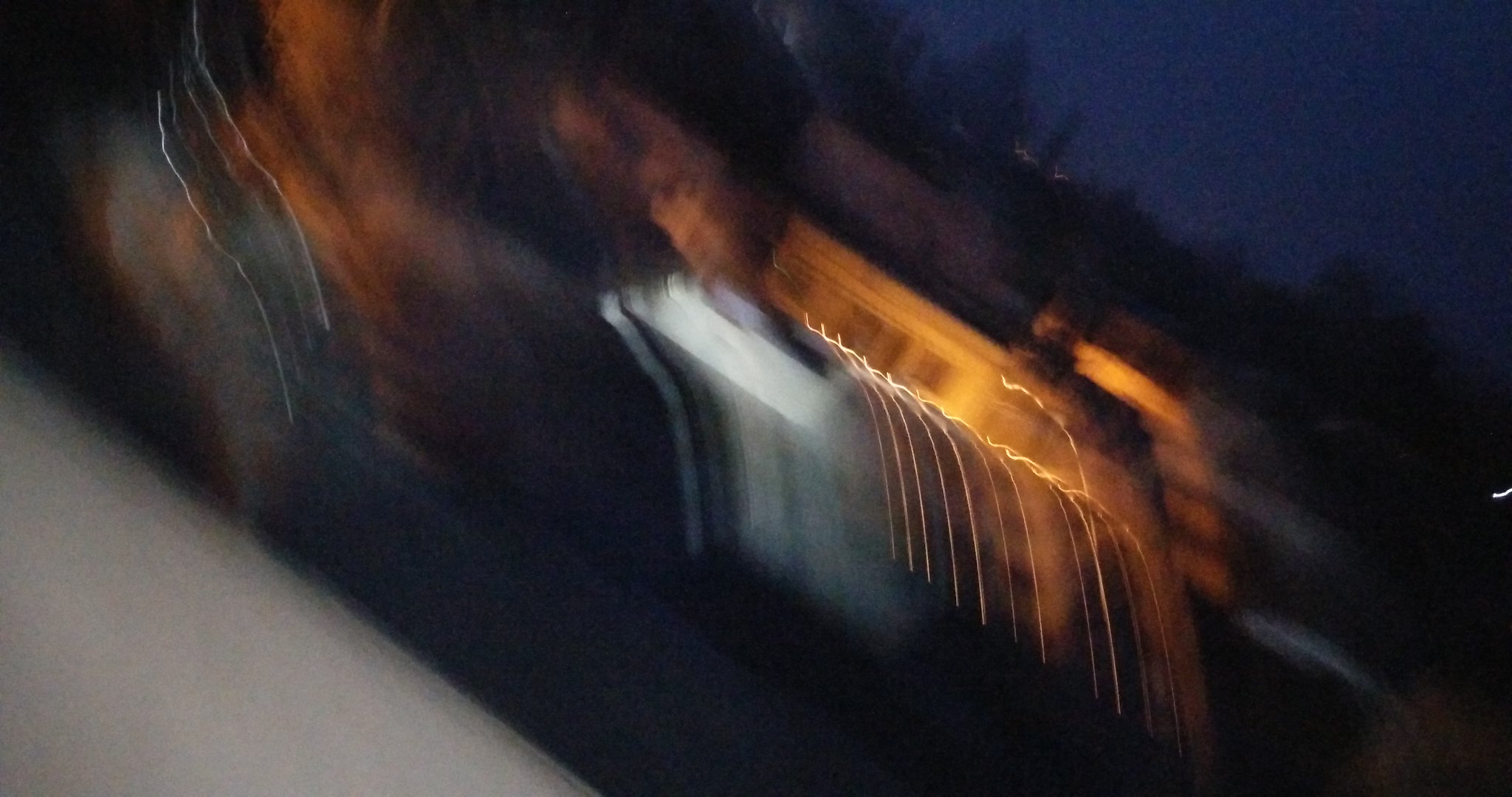This extremely blurry image, taken at night, appears to depict a city skyline viewed through a moving camera or a car window. The blurry picture shows dark indigo-blue sky occupying the upper right corner, transitioning diagonally from the left half towards the middle right. Below the sky, there's a faint tree line extending from the left center to the right center, with darkened tops. Positioned in front of the trees is the indistinct outline of a large, grayish building with a dark roof, bathed in yellowish-orange illumination. The image also features numerous streaking lines, including thick white lines resembling a waterfall and smaller yellow lines that curve downward from the center. The bottom left corner has a small, bright white triangle, adding to the confusion of the scene. Overall, the blurred streaks of light and shapes give the impression of a dynamic, distorted night view, almost like an out-of-focus oil painting or a rushed glance through a speeding car's windshield.